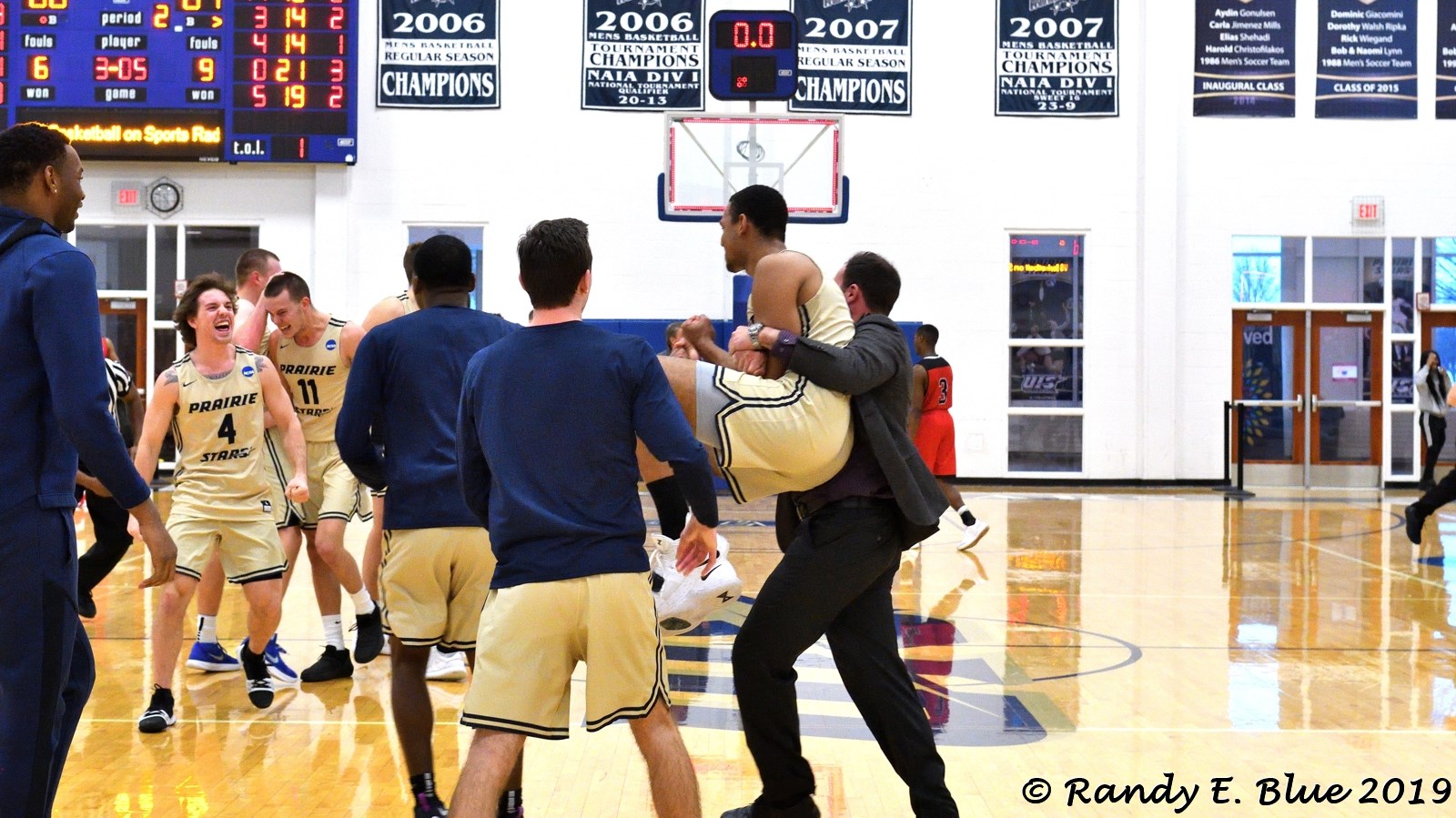In this photograph, taken by Randy E. Blue in 2019, a jubilant basketball moment is captured on a shiny gym floor. The scene unfolds on a basketball court adorned with national championship banners and a scoreboard showing neon numbers. The victorious Prairie Stars, a high school or college team in pale yellow or golden uniforms, are celebrating a game-winning shot at the buzzer. Central to the image, a jubilant coach in a suit lifts one of the players in celebration. To their right, another player, with an expression of joy and excitement, is approaching them, smiling and shouting. Visible in the backdrop are championship banners, including titles such as 2006 and 2017 men's basketball champions, and other notable achievements. The setting is an indoor nighttime event, and the overall image is a horizontal rectangle with the copyright marking in the bottom right corner. The celebration, expressions, and details make the photograph a vivid capture of a triumphant sports moment.